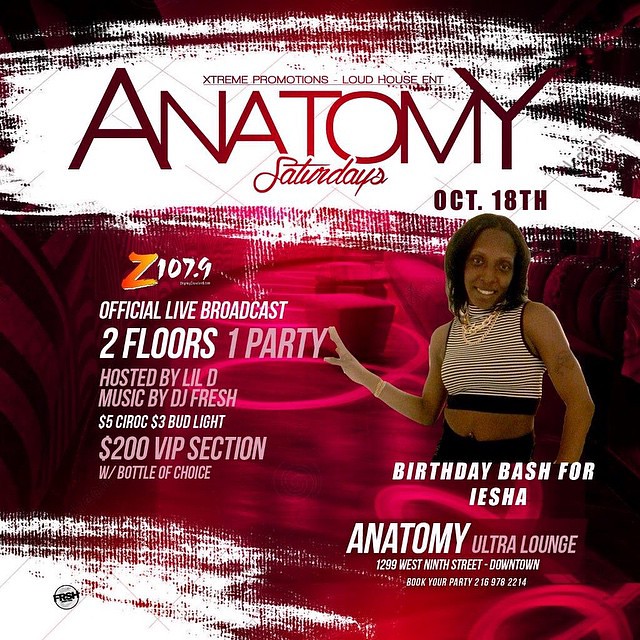This is a highly detailed and vibrant poster for an event. Set against a bold red background with black and white accents, the top of the poster announces "Extreme Promotions" and "Loud House Entertainment," celebrating "Anatomy Saturdays" on October 18th. On the left side, it details an "Official Live Broadcast" by Z107.9 featuring "Two Floors, One Party," hosted by Lil D with music by DJ Fresh. Special offers include $5 Ciroc, $3 Bud Light, and a $200 VIP section with a bottle of choice. 

On the right side of the poster, there is a striking image of a smiling woman with dark skin, adorned with gold necklaces, a black and white crop top, and black hip-hugger pants. This section highlights a "Birthday Bash for Aisha" at Anatomy Ultra Lounge, located at 1299 West 9th Street Downtown. Information for booking your party is also provided: call 216-976-2214. The cohesive design, with prominent fonts in pink and white, ensures the details of this lively event are both eye-catching and memorable.